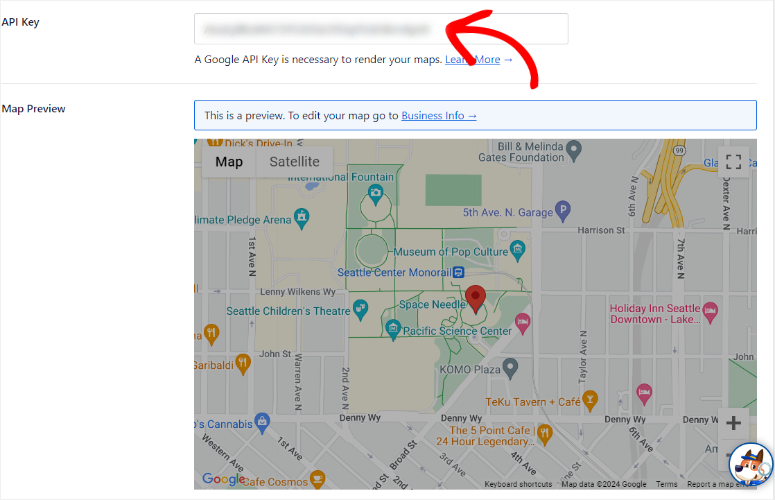The image shows a window with a thin gray border. In the top left corner, "API key" is written in black font using a basic sans-serif typeface. To the right of this text is an editable field, with the entered text blurred out for privacy. A red arrow points to this blurred text and also directs attention to a light blue rectangle with a dark blue border, which contains a message in black font: "This is a preview period to edit your map go to," followed by an underlined blue link labeled "business info." Another part of the message beneath the blurred area states, "A Google API key is necessary to render your maps," accompanied by an underlined blue link that says "learn more," with an arrow pointing to the right of the link.

Below this header, there is a detailed map. Various roads are marked in white, and several map pins of different colors indicate various locations. Aqua pins signify general points of interest, orange pins indicate food locations, blue pins highlight shopping areas, a red pin denotes the user's current location, and pink pins represent lodging options. 

In the top left corner of the map, two rectangles are separated by a gray border. The left rectangle, marked "map" in bold black text, contrasts with the right rectangle labeled "satellite," which is not bolded. 

On the far right, there is a white square containing a pattern of gray points that form a square from the top left to the bottom right. At the very bottom right of the map, there is a white circular icon with a blue border featuring a cartoon dog wearing a hat and looking through a magnifying glass.